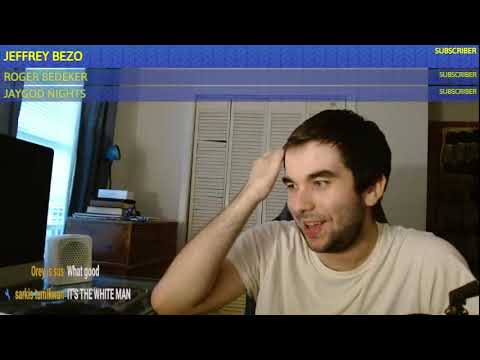The image depicts a vintage-looking screenshot of a YouTube live stream featuring a man seated at a desk in his home office. At the top of the image, there are three names listed in yellow uppercase text on blue stripes: "Jeffrey Bezo, subscriber," "Roger Bedecker, subscriber," and "Jay God Knights, subscriber." The background shows a white wall and a white closet door directly behind the man. To the far left, there's a black TV screen beneath an open window with gray blinds, allowing natural light to filter through. Just to the left of the man, a brown table holds several books and a lamp. The man, off-centered to the right, wears a white t-shirt; he has dark hair and light stubble, and he is seen smiling with his mouth slightly open, seemingly amused by something on his screen. He has his left hand reaching up toward his hair while looking leftward at the screen. The bottom left corner features a chat reading, “What good,” followed by, “It’s the white man.”